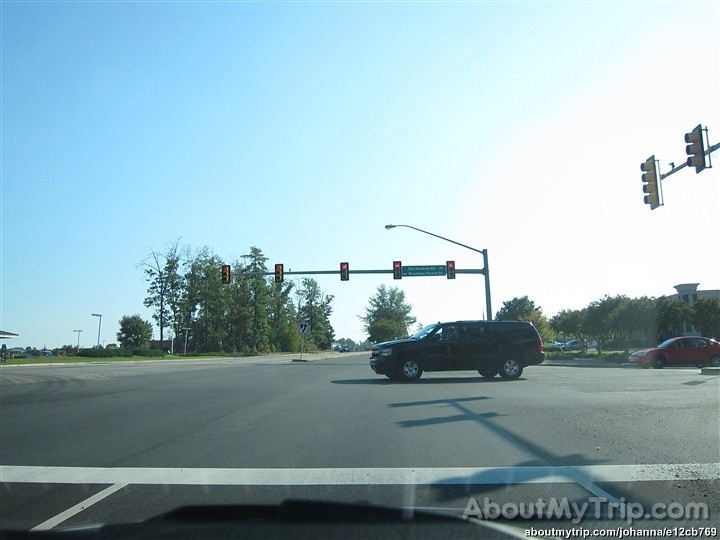The image depicts a busy intersection viewed from inside a car waiting at a red light. Directly ahead, in the lane, is a black SUV, with a red sedan positioned behind it. To the left, there is a flow of cars moving horizontally from right to left. Dominating the scene, a tall pole rises with five red traffic lights and a street lamp mounted at the top. On the right side of the scene, additional traffic lights serve vehicles traveling from left to right. Beyond the intersection, a stretch of grassy areas and trees can be seen, alongside a building and a parking lot to the right. The detailed urban landscape highlights the complexities of city driving.